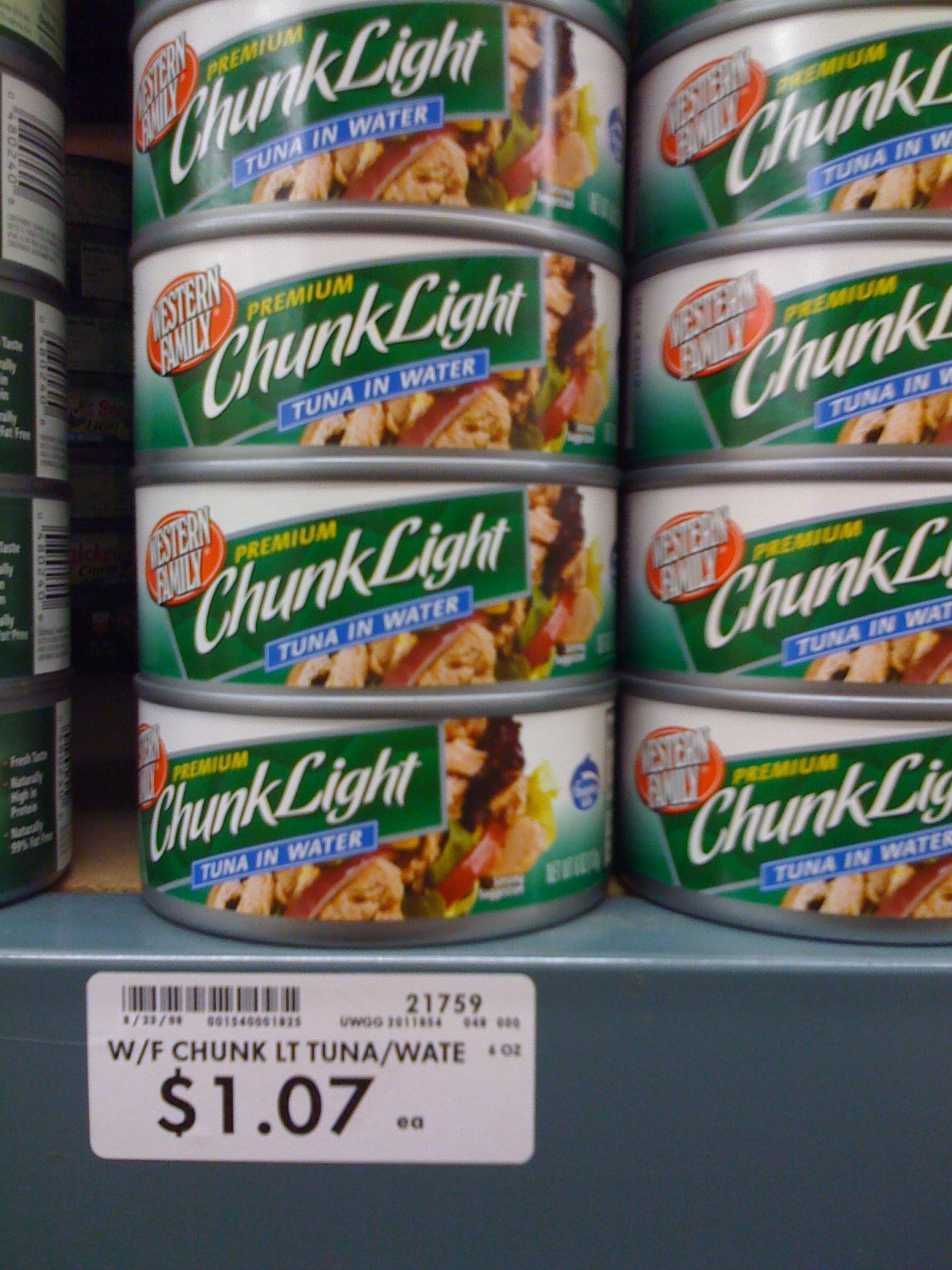The photograph captures a retail grocery store shelf stocked with Western Family Premium Chunk Light Tuna in Water. The cans, predominantly green and white, prominently display a tuna salad image with red onions and green lettuce. The visible shelf, made of dark gray steel, supports multiple stacks of tuna cans. While the forefront shows four fully-visible cans, partial views of additional cans suggest these stacks may reach up to seven cans high. A white label attached to the shelf edge reads "W/F chunk LT tuna/WATER" and lists the price as $1.07 each, accompanied by a barcode and the number 21759 for scanning purposes.